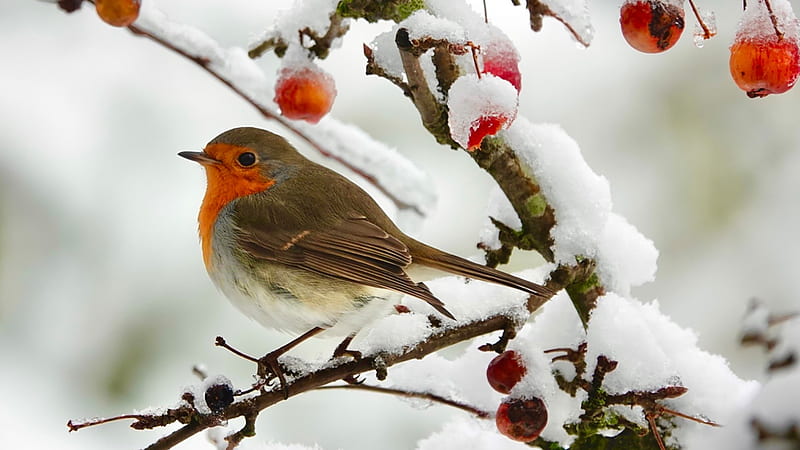A vibrant, plump bird is perched on a snow-covered branch in this detailed winter scene. Centered slightly to the left, the bird stands out with its striking plumage: a dark grey back, wings, and tail, contrasted by an orange-reddish face and neck, a white belly, and a long brown tail. The bird's black beak and feet add sharp details to its round silhouette. Around the bird, the tree branches extend outward, laden with thick snow and clusters of glossy red berries, some of which have white accents due to the snow. The blurred background features smooth transitions of gray and off-white, making the bird and the snow-draped branches the clear focal points. Predominant colors in the image include brown, white, shades of blue, orange, and red, creating a beautiful and vivid winter tableau. No text is present in the image.